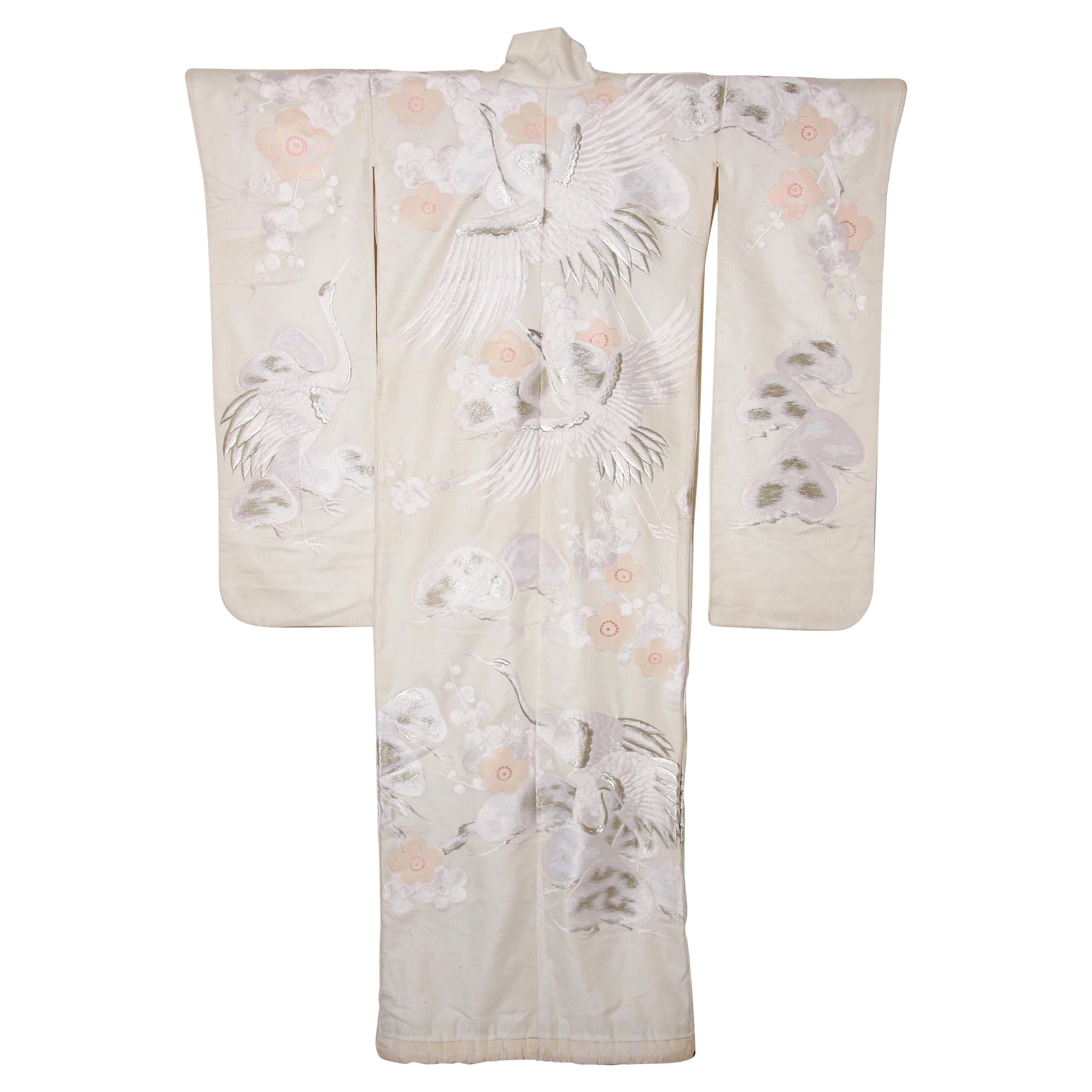This photograph showcases a vintage cream-colored kimono set against a pristine white background, reminiscent of a product image one might find on retail websites. The kimono, displayed flat on a rectangular hanger, creates a square appearance with long sleeves draping on both sides and a central body featuring a collared neckline akin to a turtleneck.

Adorning the kimono are intricate designs that include cranes and flowers. Central to the garment's decoration are two large cranes positioned amidst clouds, with one appearing to soar above, and another standing, creating a serene scene. Surrounding these cranes are pink, white, and muted peach flowers, extending onto the right sleeve and further accentuating the ethereal landscape depicted across the fabric. Towards the bottom, additional elements like stones or jellyfish motifs blend with the floral and avian designs, enhancing the kimono's vintage aesthetic and overall harmony.